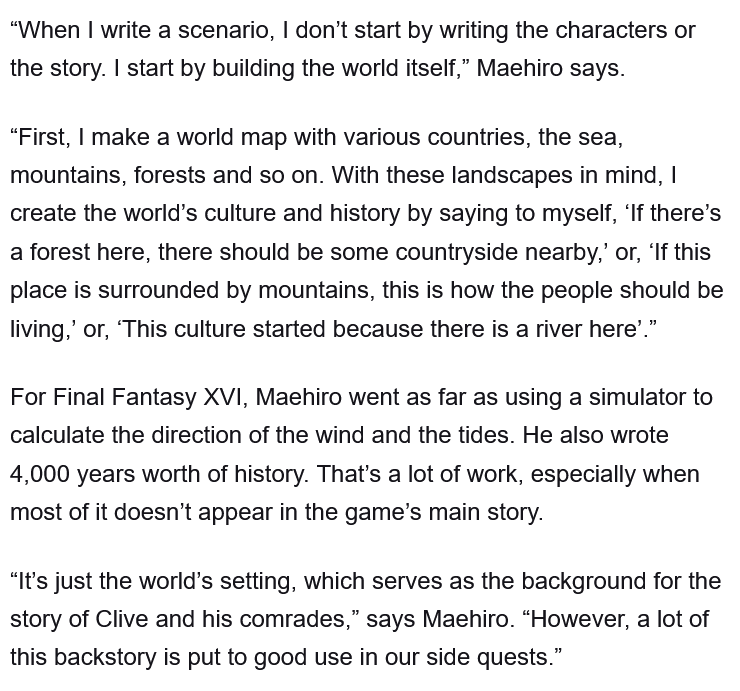This image features black text on a plain white background, resembling a page from a digital book. The text is an insightful quote detailing the creative process of a writer, referred to as Mihiro or My Hero. It begins with: "When I write a scenario, I don't start by writing the characters or the story. I start by building the world itself." Mihiro explains that the first step is to create a world map featuring various countries, seas, mountains, forests, and other landscapes. He elaborates that these landscapes inform the world's culture and history, forming a narrative that, for example, a forest should have nearby countryside or a river would give rise to a particular culture. The process of world-building for Final Fantasy XVI was meticulous, involving the use of a simulator to calculate the direction of the wind and tides, and the creation of 4,000 years' worth of history. Although much of this detailed backstory doesn't appear in the main story of Clive and his comrades, it enriches the game's setting and is utilized in the side quests, thereby enhancing the overall immersive experience.